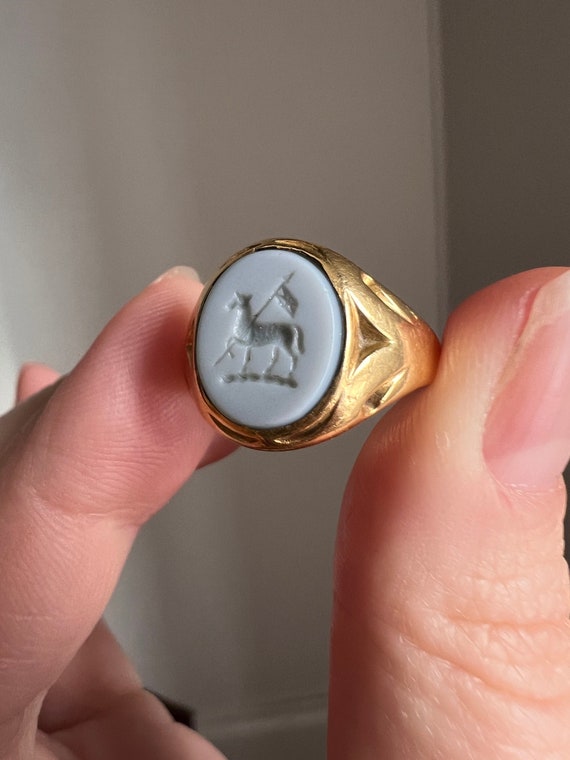The photograph is a close-up of a person’s thumb and index finger holding a golden ring. The gold ring features an intricate design on its face, which seems to be a light gray or ivory base. The central emblem on the ring depicts a horse-like animal walking on three legs while holding up a flag with its raised front left leg. The ring itself is somewhat large, suggesting it may be a men’s ring, and has additional etchings along the band that resemble diamond shapes with two lines. The image is highly zoomed in, highlighting the fingers—especially the long index finger—while the person's pinky finger is faintly visible in the background. The backdrop consists of plain, white walls, emphasizing the ring and hand as the primary subjects of the photograph. Overall, the detailed close-up focuses on the gold ring with its symbolic engraving, framed by the hand holding it against a minimalistic setting.